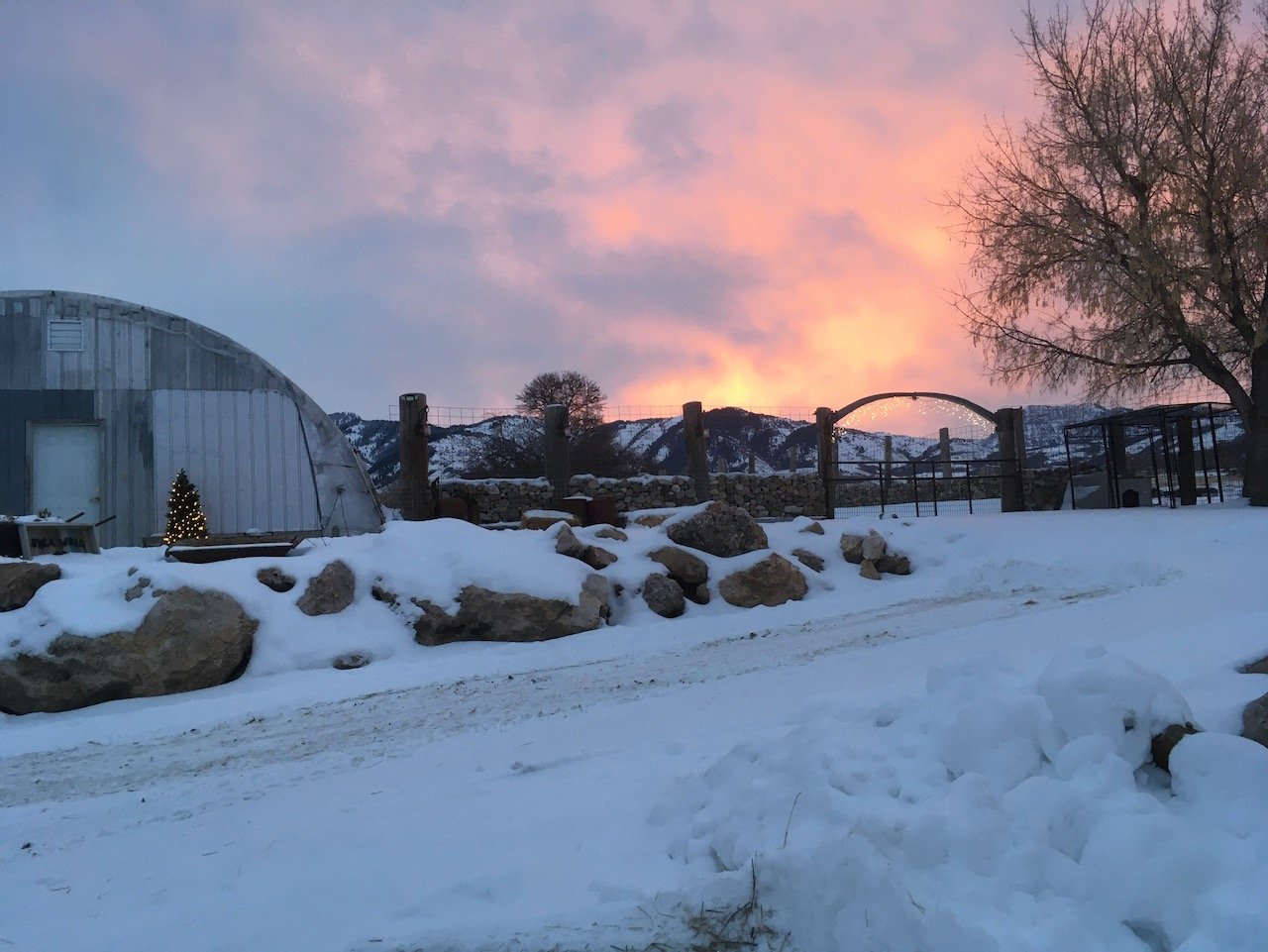The image captures a serene winter sunset or sunrise at a snow-covered ranch. Dominating the left side of the frame is a Quonset hut-style metal hanger with a distinctive flat-front door. In front of this hanger stands a lit Christmas tree, approximately three and a half feet tall, adorned with white lights. The foreground reveals a snow-covered driveway bordered by rocks, also blanketed in snow. To the right, a fence is visible, constructed from wooden posts with a wire grid between them, and some sections stacked with thin-cut logs. Atop this fence, there's an archway decorated with white Christmas lights. A massive tree stands to the right, framing the image, and in the background, majestic, snow-covered mountains rise against a beautifully colored sky painted in hues of pink, orange, purple, and peach. The sky and cloud formations hint at an enchanting sunset or sunrise, casting a warm, glowy light throughout the scene.